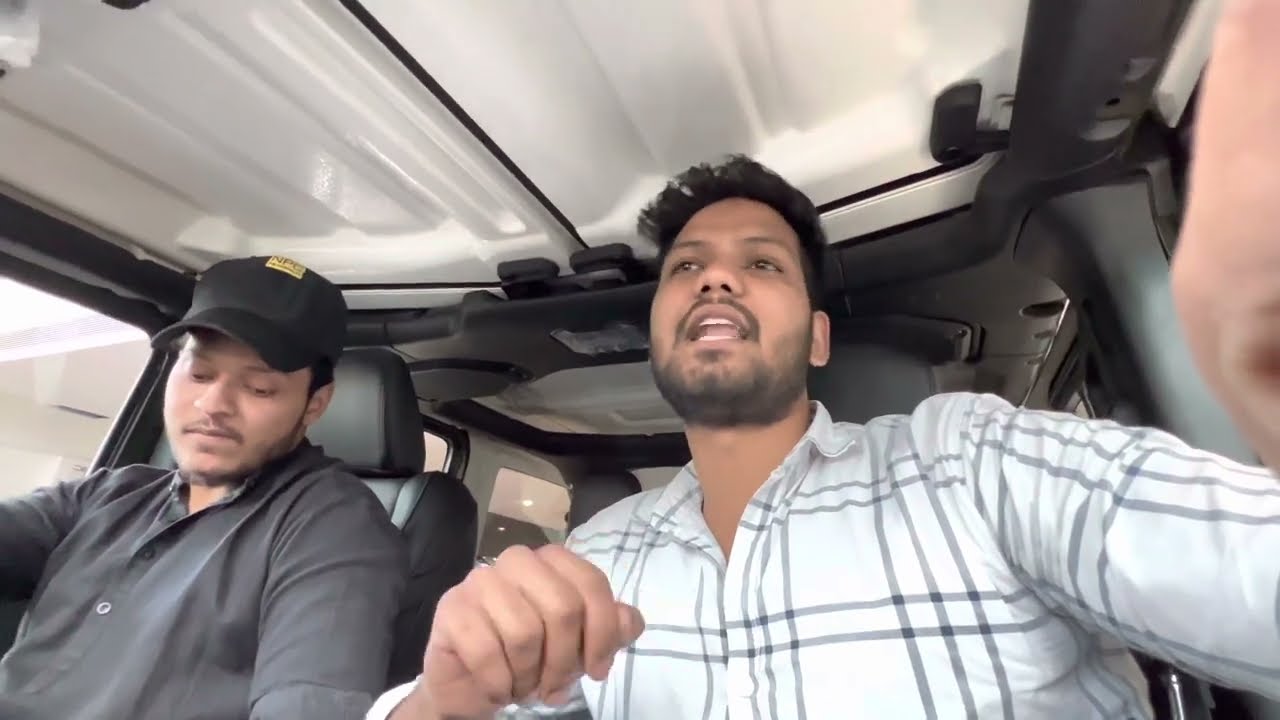The image captures two men of Indian descent inside a vehicle, likely a cargo or transport van. The focus is on the man in the driver's seat, who has a short, gelled-up black hair and a dark beard extending into a pronounced handlebar mustache. He appears to be singing or speaking, with his mouth open and teeth apart, revealing his tongue. He is dressed in a white button-up shirt with grey stripes. The man in the passenger seat, who looks similar to the driver and could be a brother or friend, is wearing a dark grey button-up shirt and a black hat with a gold label or patch on the front. He has a thinner mustache and beard and is looking downward. The setting is bright and illuminated by natural daylight, suggesting the image was taken during the day. Part of the driver's hand is visible in the shot, indicating he might have taken the photo himself.